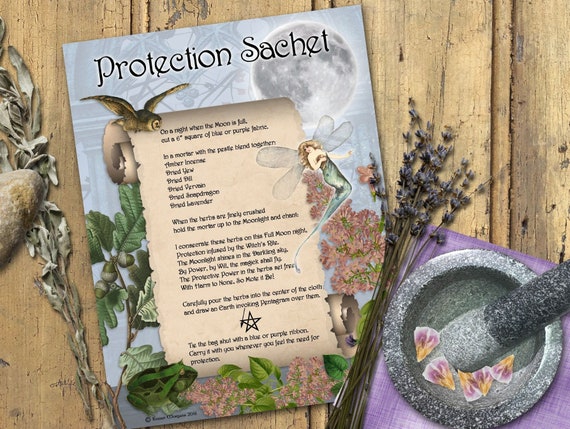The image portrays an art project laid out on a rough, natural wood table. Central to the composition is an instruction sheet titled "Protection Sachet." This sheet features an illustrated scroll adorned with a whimsical fairy in a green dress, a small brown owl at the top, a green frog at the bottom, along with pink flowers, green leaves, and a celestial symbol, most likely a Wiccan star, enhancing its earthy, mystical theme. The instructions on the scroll are too small to read but are related to creating an herbal protection sachet, possibly invoking magical or Wiccan traditions under a full moon.

To the right of the instruction sheet sits a stone or metal mortar and pestle filled with flower petals, hinting at the preparation of ingredients for the sachet. Nearby are sprigs of herbs and tiny purple flowers, suggesting additional components for the project. A purple tapestry occupies the bottom right corner of the table, adding a touch of color and texture to the scene. Overall, the image is carefully curated, blending natural elements and mystical symbols to create an intriguing, earthy ambiance.